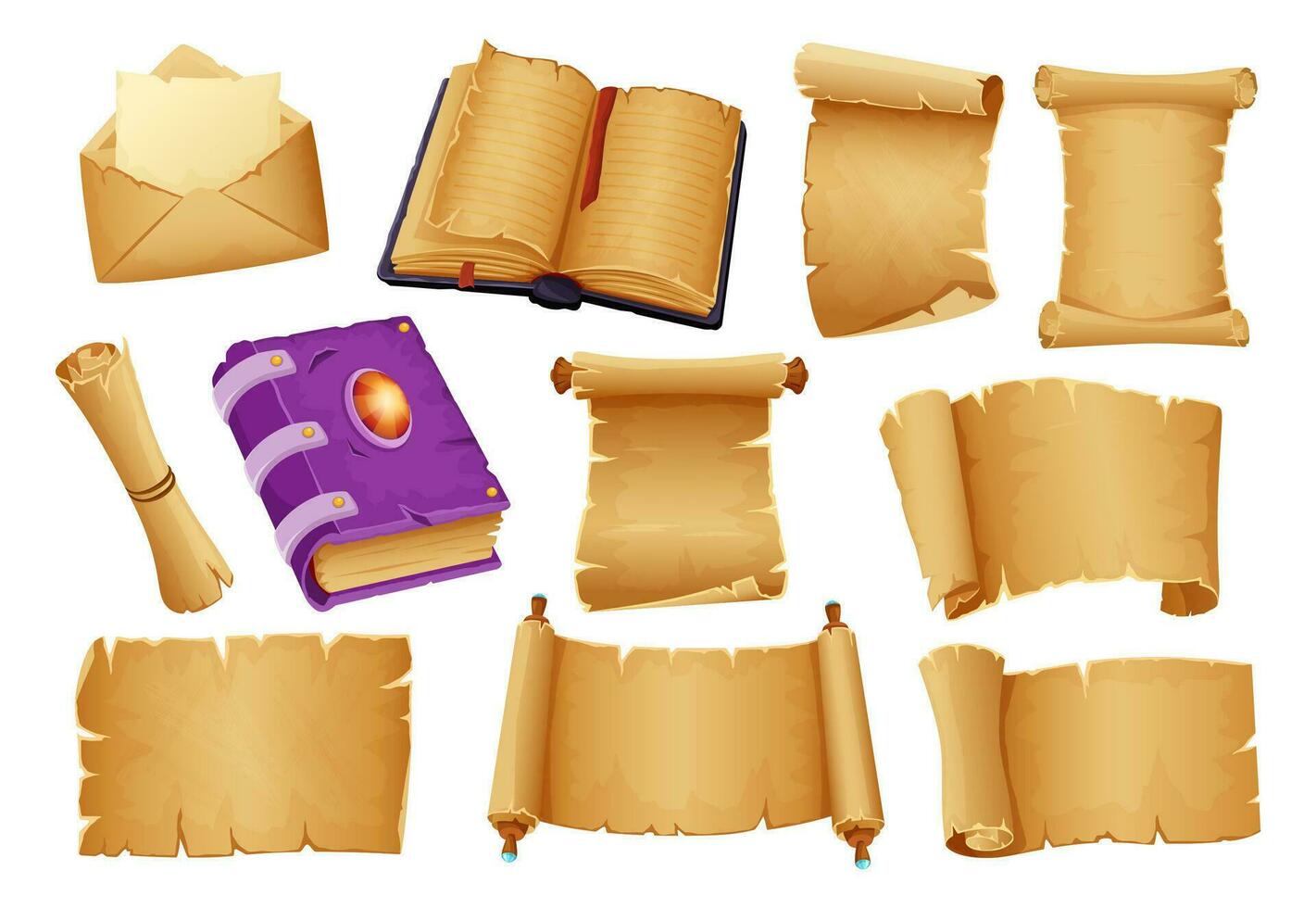This digital image on a white background features a meticulously arranged collage of medieval-inspired paper objects and books. The primary color theme is brown, reflecting an aged, parchment-like aesthetic. In the upper left corner, an open brown envelope reveals a lighter brown piece of paper peeking out. Immediately to its right, an open book with a black cover displays lined pages, anchored by a red ribbon bookmark. Beside it, two tattered, blank scrolls add a rustic charm with their jagged edges, one slightly curled at the top and the other rolled at both ends.

Centering the composition, a trio of items includes a rolled-up brown scroll, a distinguished hardcover book in purple adorned with an ornate orange gemstone and three silver bands, and another aged scroll, this one vertically extended and rolled at the top around a wooden peg. Flanking this central row are horizontally and vertically positioned scrolls, further contributing to the image's symmetrical balance.

On the bottom row, three more scrolls complete the collage. The one at the far left lies flat and unmarked, while the middle scroll mimics the classical look with both ends rolled around wooden pegs. The final scroll unrolls from the left side, tapering off flatly to the right.

The collective display, though digitally rendered, authentically mimics various paper forms from ancient manuscripts to scrolls, presenting a visually cohesive and evocative collection.